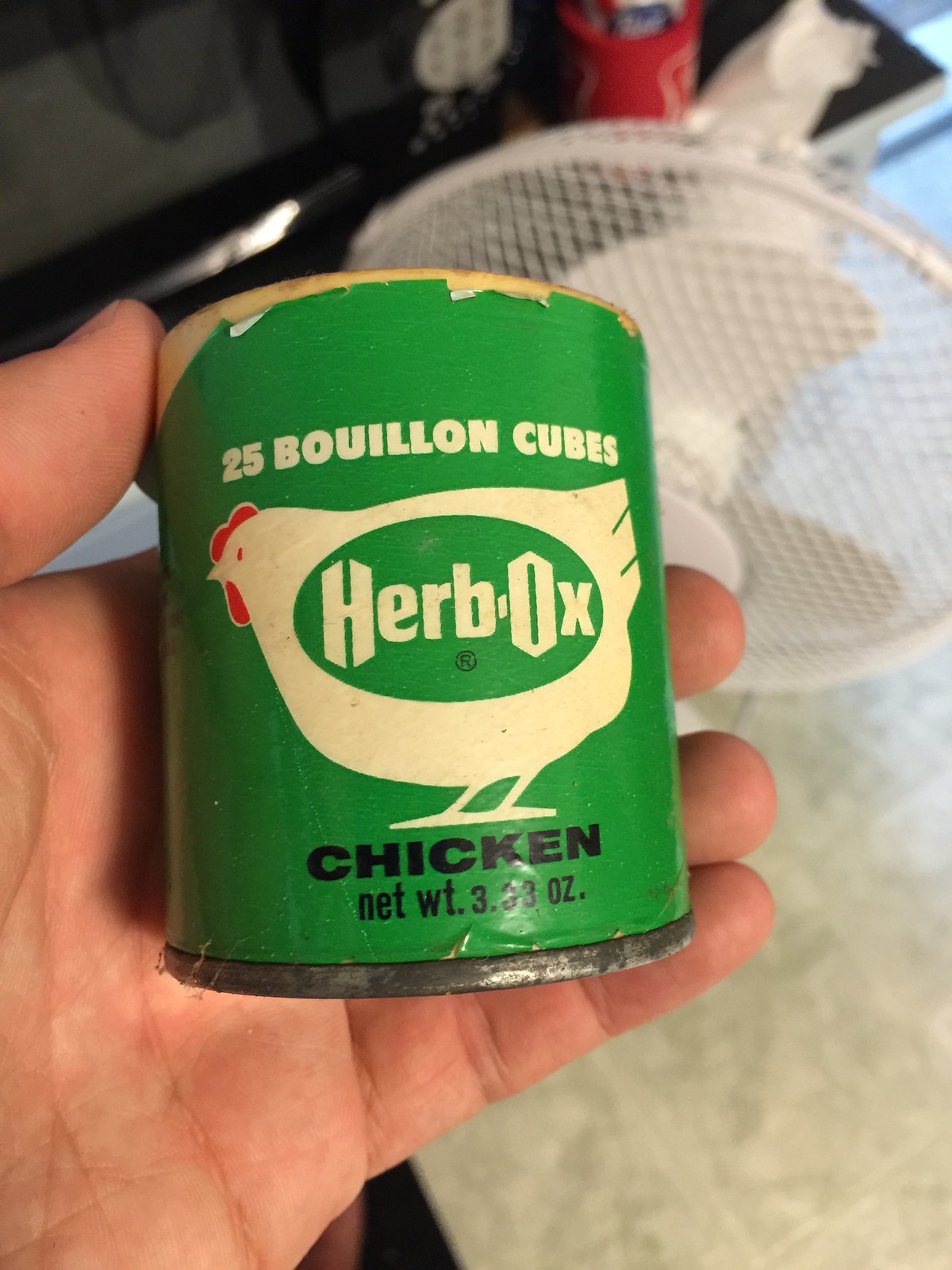A close-up image shows a hand holding a worn green can of Herbo Ox Chicken Bouillon cubes upright towards the camera. The can prominently features a white chicken with a red comb and eyes. Clearly labeled, the can contains 25 bouillon cubes in small white letters, with "Herbo Ox" in the center in white lettering, and "chicken" in black below it. The net weight of 3.5 ounces is also displayed. The hand gripping the can reveals four fingers, suggesting the can is cradled in the palm. In the blurred background, a small white fan is visible, possibly placed on a white table or the floor, further emphasizing the focal point on the aged can.